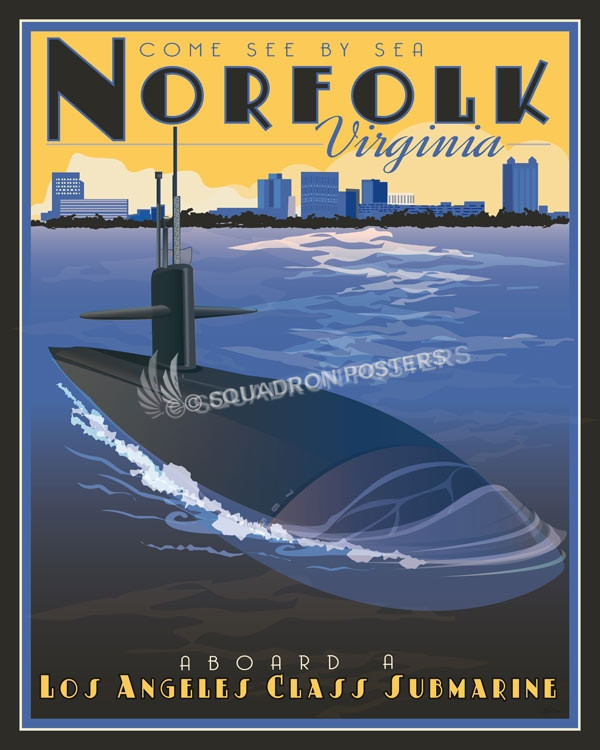This vintage-style poster, created by Squadron Posters, vividly advertises Norfolk, Virginia. Dominating the scene is a Los Angeles-class submarine cutting through the blue ocean waves, with white caps forming around its prow. The city's skyline serves as a backdrop, contrasting with the expansive water stretching in the foreground. At the top, large black letters on a yellow background read, "Come See by Sea," promoting Norfolk's maritime allure. The phrase repeats in smaller letters, bolstering the call to explore the city's naval attractions. Beneath the image, bold text further emphasizes the unique opportunity to visit "Aboard a Los Angeles Class Submarine." The artwork is framed with a black border, complemented by a thin white strip and a wider blue strip, enhancing its eye-catching appeal.